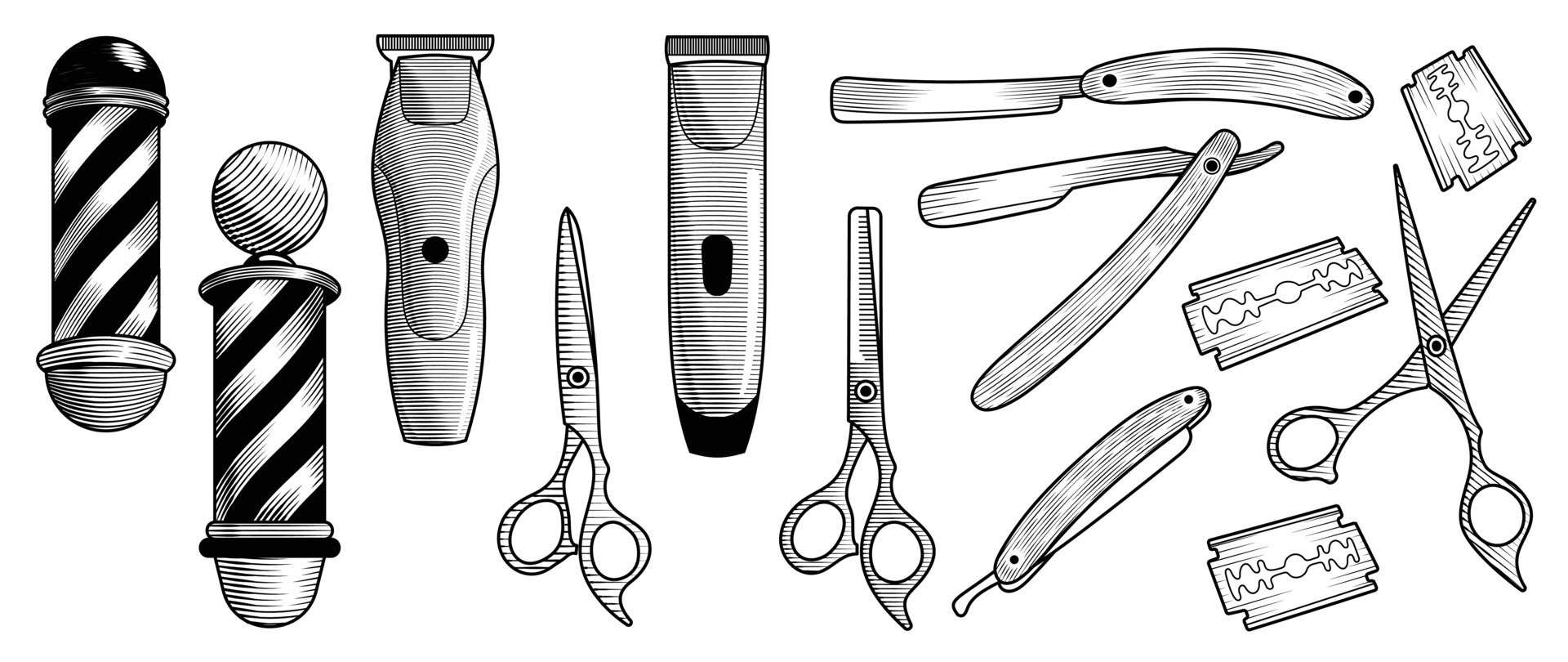The image is a detailed black and white line drawing showcasing various tools and elements typically found in a barbershop. On the left side, there are two classic barber poles with diagonal stripes, one with a black top and the other with a white top. Next to the poles, there is an electric hair clipper followed by a pair of barber scissors and another type of electric razor. Moving further to the right, there are more straight razors depicted in three positions: fully open, half-folded, and completely folded, reminiscent of a jackknife's design. Below these razors are three double-edged razor blades commonly used in safety razors. Close to the blades is another pair of barber scissors, specifically thinning shears, which are used for detailed work and have fine, pointed tips. The illustration is rendered with intricate fine lines and varying shades of grey, capturing the essence and detail of each barbershop tool vividly.